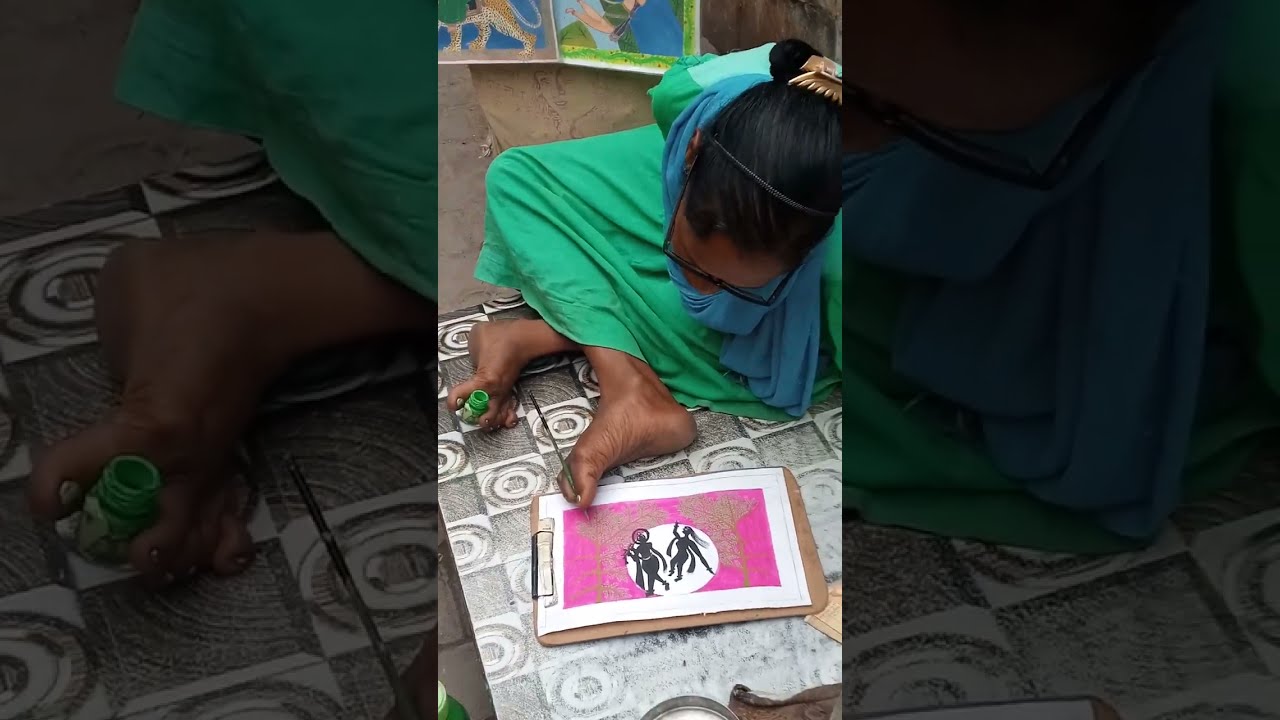In this captivating image, a young girl with black hair tightly pulled back, dressed in a green dress paired with a blue scarf wrapped around her neck, is seated on a tiled surface. Her legs are crossed in front of her, revealing her feet. Remarkably, she is using her feet to create art on an 8.5 x 11 sheet of paper secured to a clipboard. Her left foot grips a green ink bottle between her toes, while her right foot holds a pen or paintbrush, with which she draws on the paper. The artwork features a large pink square with a white circle inside it, depicting two dark silhouettes against a background that resembles the moon. On a closer look, elements such as a tree are discernible. Above the girl, two completed paintings are displayed on the wall. The left side of the image offers a zoomed-in view of the green ink bottle. The right side, however, remains cloaked in darkness, leaving only faint hints of the blue scarf and green dress. This touching scene highlights the girl's remarkable dexterity and creative spirit.